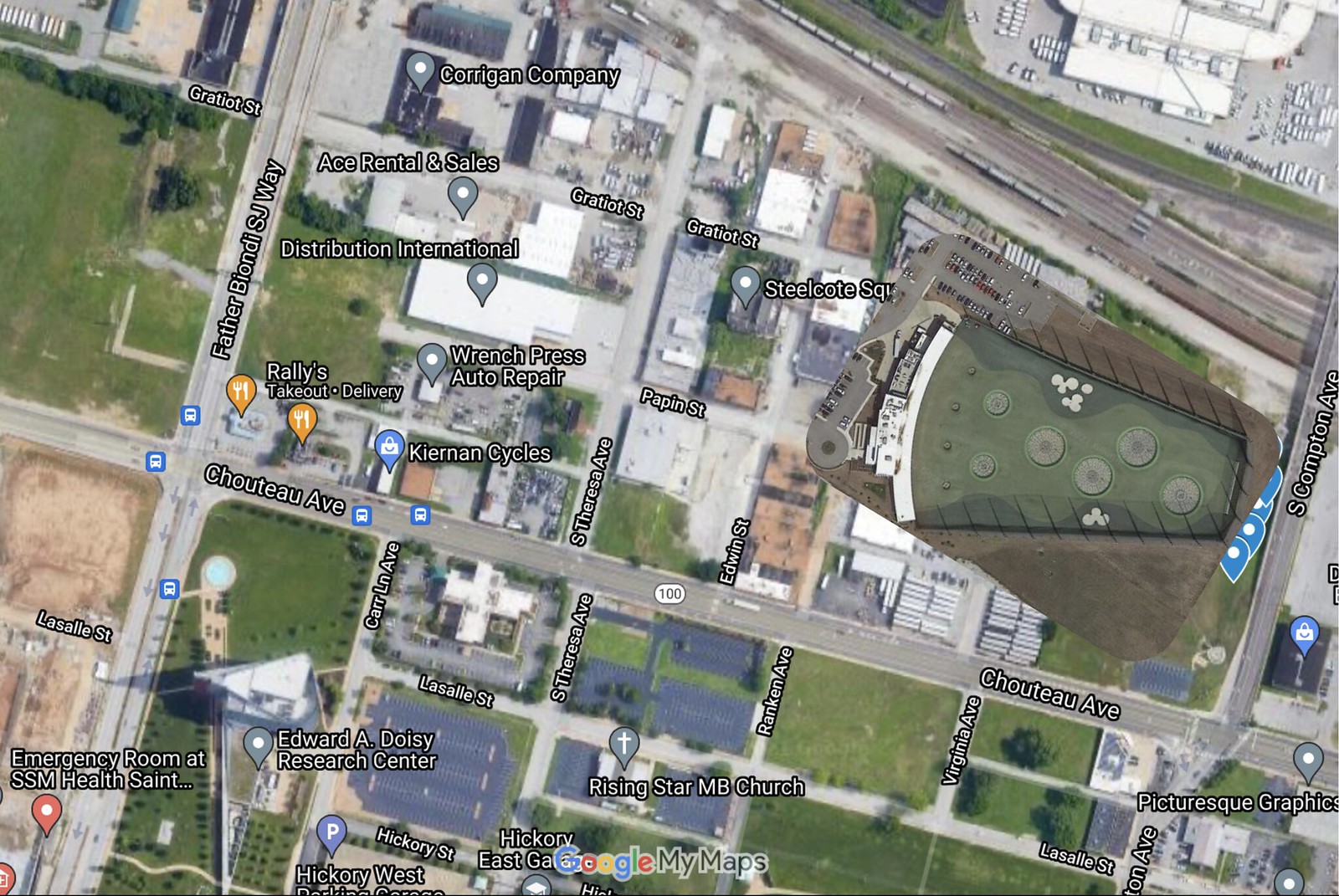This image is an overhead view from Google Maps, showcasing a detailed layout of a city area with clear satellite imaging and labeling. The view provides a bird's eye perspective, prominently featuring various roads, landmarks, and businesses. Key roads include Chouteau Avenue running east to west, and intersecting it north to south are Father Bondi S.J. Way and South Compton Avenue. Other streets visible are Virginia Avenue, Liddell Street, Pepton Street, South Teresa Avenue, and Edwin Street. 

Landmarks and establishments mapped out in this image include the Emergency Room at SSM Health St. Edward A. Doisy Research Center, Rising Star MB Church, Rally's Takeout Delivery, Ace Rental and Sales, Distribution International, Corrigan Company, Ranch Press Auto Repair, Picturesque Graphics, Keenan Cycles, and Steel Cut Square. The image also shows parking areas with cars and patches of grassland, adding to the comprehensive urban detail captured in this Google My Maps view.